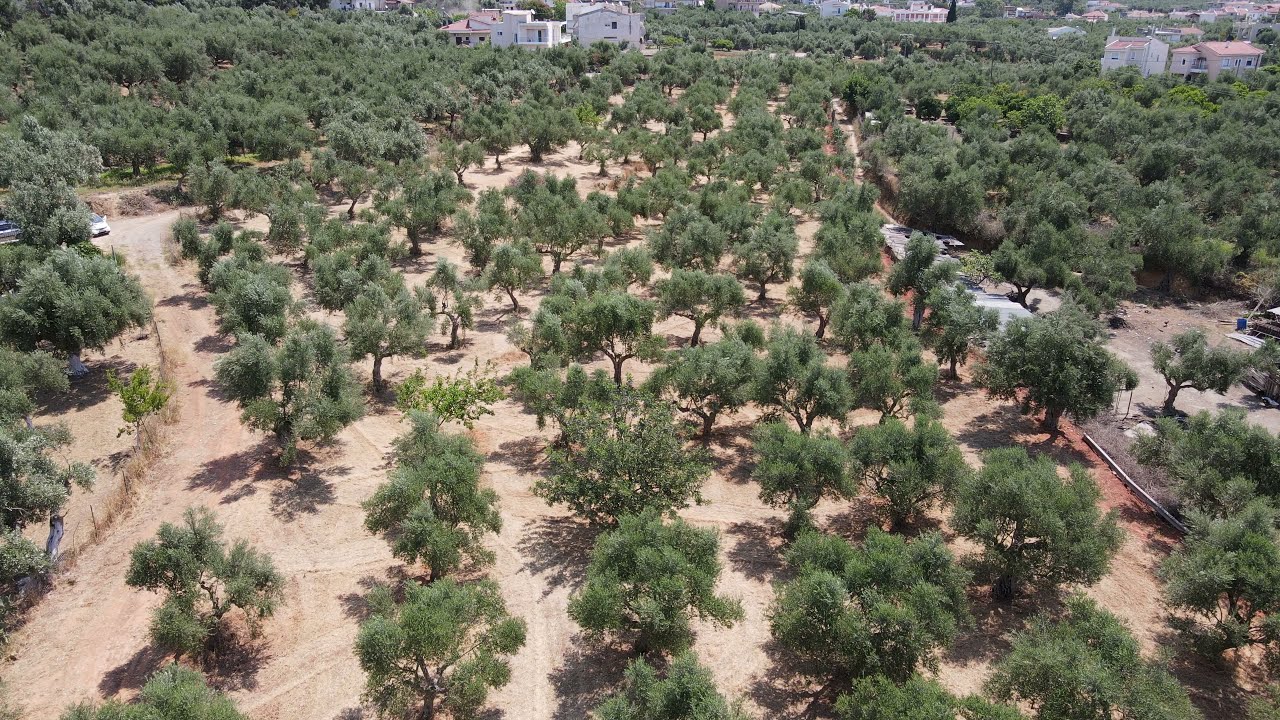The image captures a sunny scene of a large, dry, wooded area featuring a variety of deciduous trees. The earth throughout the scene has a parched, reddish-sand texture, with patches of dry dirt intermingled with more sandy hues. A dirt road traverses the left side of the image, creating a visible pathway amid the sparse spacing of the trees. These trees are arranged in strategic rows, set on a lower level than the surrounding land, with their dry undergrowth clearly visible.

In the background, a cluster of houses appears spread out across the rear center and right portions of the image. The structures vary in size but generally consist of a couple of stories. Notably, a prominent house in the center background sports a distinct red-toned roof. Similarly, another building with a red roof is observed at an angle towards the front of the house on the far right side. There’s also a small white car parked towards the upper left corner near an area with a hint of grass. The backdrop offers a mix of additional houses, enriching the rural yet somewhat residential atmosphere of the scene.